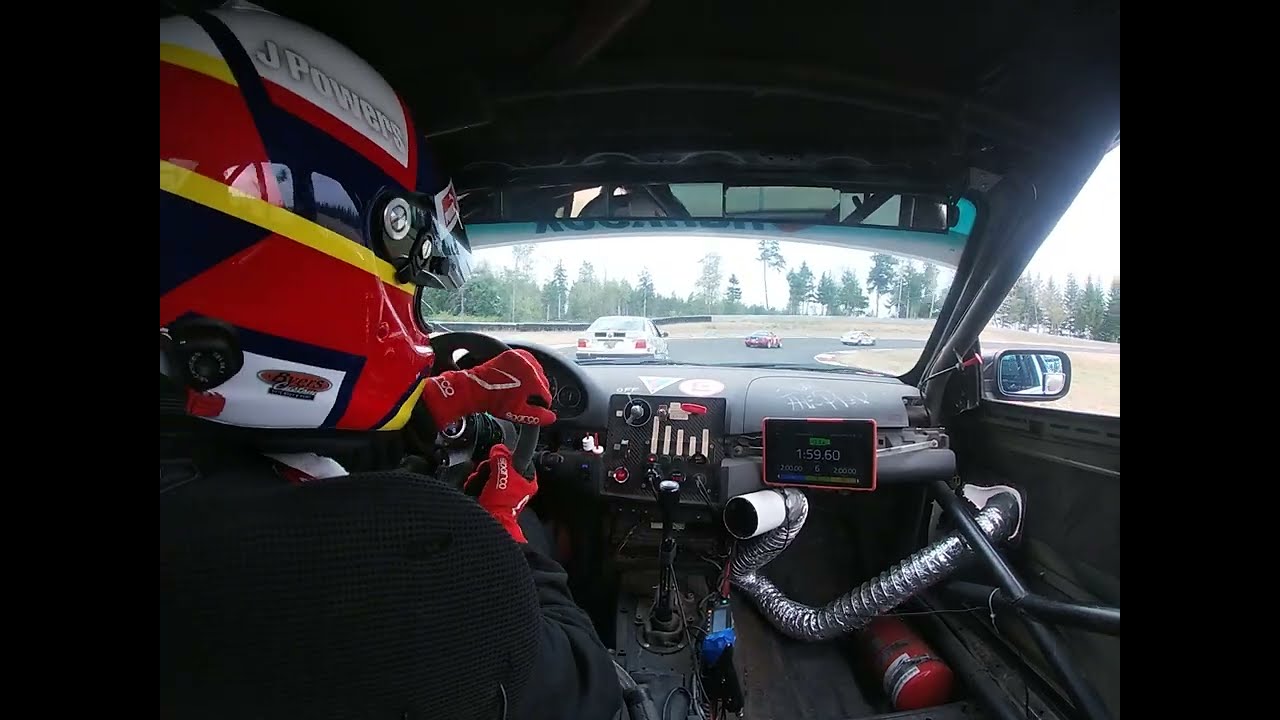The image captures the interior of a race car from the perspective behind the driver's seat, framed by thick black vertical borders on each side. The car’s interior is predominantly black, and within the top-left corner of the image, the driver’s helmet is partially visible. The helmet, emblazoned with the name "J Powers" in white font, features an eye-catching design with colors of bright red, navy blue, yellow, and white. The driver, dressed in a black jacket, is gripping the black steering wheel with red and white gloves. To the right inside the car, there are several contraptions and two screens that display vital information; one of the screens, a digital speedometer, indicates the car is traveling at 159 miles per hour. Below the smaller screen, a white gadget with a silver pipe is visible. Through the car's windshield, the race track and several other cars ahead are clearly seen, with three cars immediately in front and trees lining the background, adding depth to the racing scene.